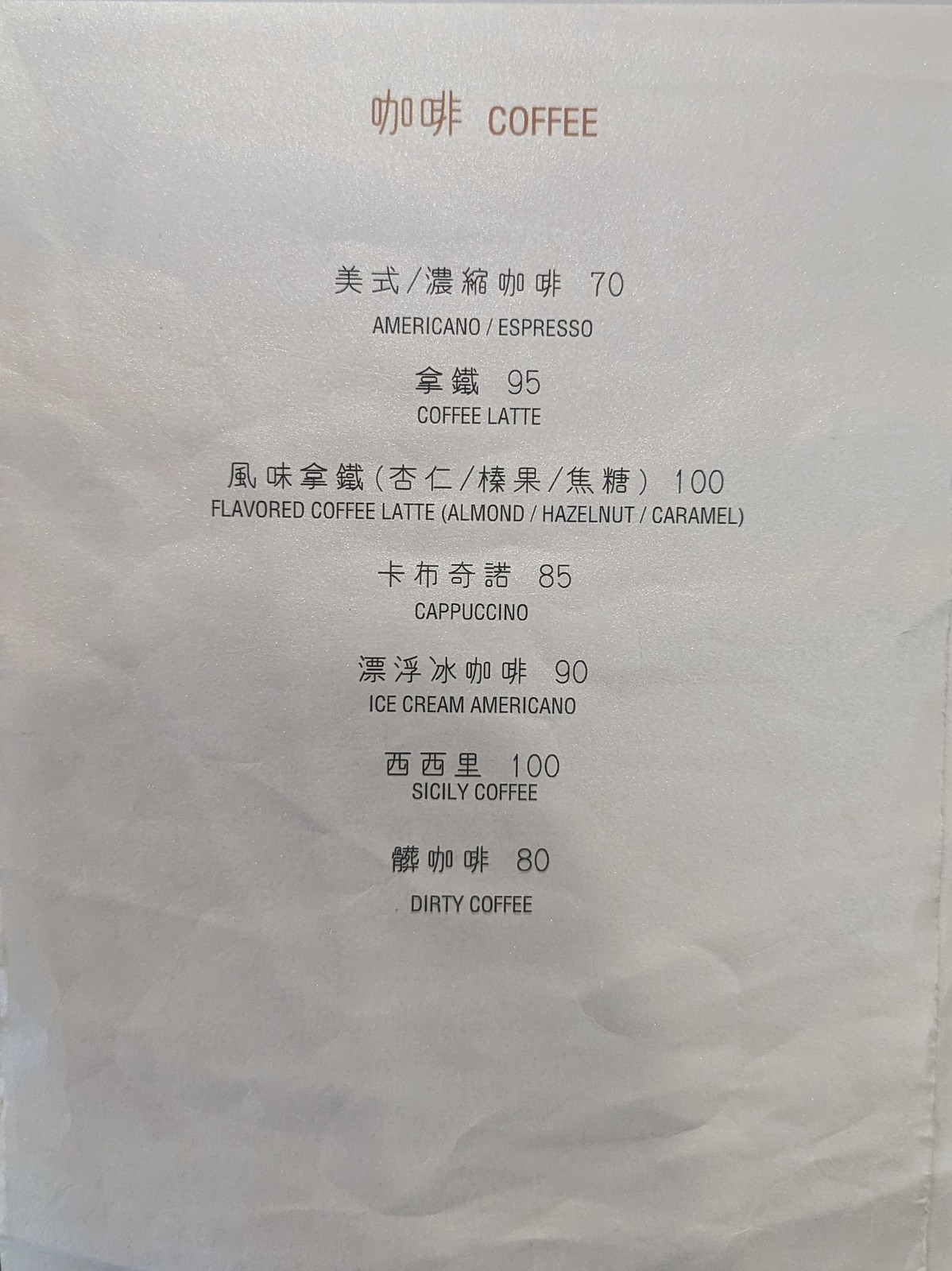This photograph features a white, slightly wrinkled piece of paper, adorned with red and black text as well as symbols resembling Chinese or Japanese characters. At the top of the page, in a reddish-orange font, are symbols followed by the word "COFFEE." Below, in black font, the menu items are listed:

- "70 Americano / Espresso" followed by symbols
- "95 Coffee Latte" followed by symbols
- "100 Flavored Coffee Latte (Almond / Hazelnut / Caramel)"
- "85 Cappuccino" followed by symbols
- "90 Ice Cream Americano" followed by symbols
- "100 Sicily Coffee" followed by symbols
- "80 Dirty Coffee"

The sheet exhibits some shadowing and light reflection, particularly towards the bottom, adding to its textured appearance. The text is clearly legible despite the paper's creases and subtle light play.